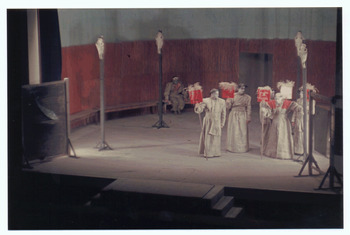The image displays a scene from a stage play, slightly fuzzy and small in size, featuring five people dressed in long, light-colored robes, possibly white or beige, and adorned with staffs topped with small red banners or signs, with a hint of straw at the top. The stage setup includes a curved bench along a semicircular back wall, with an entranceway in the center. The wall is divided into a burgundy lower half and a green upper half, possibly suggesting an old or outdoor setting. Four posts with white additions and floor-standing torches provide illumination, casting light on the stage, which remains the focal point. In the background, near the entrance, a person dressed in military-like attire is seated, adding to the drab, tan and olive color scheme of the scene. The overall atmosphere suggests a somber or protest-like gathering, with the figures on stage giving an impression of historical or Victorian era characters, possibly in a prison yard setting indicated by the walled backdrop and the seated figure's positioning and dress.